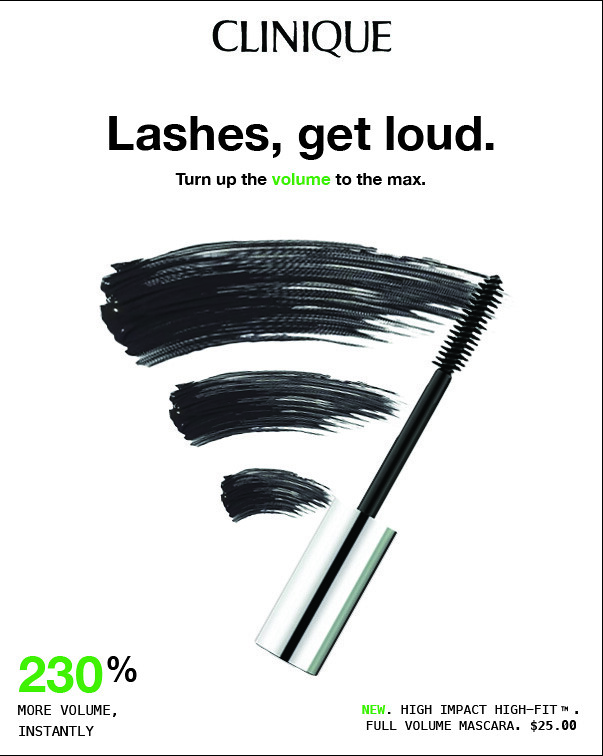The advertisement sheet features a bold black header at the top with the brand name "CLINIQUE" in capital letters. Directly below, the tagline "Lashes Get Loud" is prominently displayed in black text. The subheading further entices with, "Turn up the volume to the max," where the word "volume" is uniquely highlighted in green.

Central to the design is an image of a lash wand with a white cylindrical handle, transitioning into a black rod ending in detailed bristles. Beside the wand, three brush strokes in black demonstrate the varying intensities this mascara can achieve, with the strokes getting progressively smaller from top to bottom, indicating full, two-thirds, and half bristle usage.

In the lower left corner, a bold green "230%" stands out, followed by black text declaring "more volume instantly." The lower right corner features the word "new" in green, paired with a detailed description in black: "High-impact, high-fit, full-volume mascara." The price is clearly marked as $25.